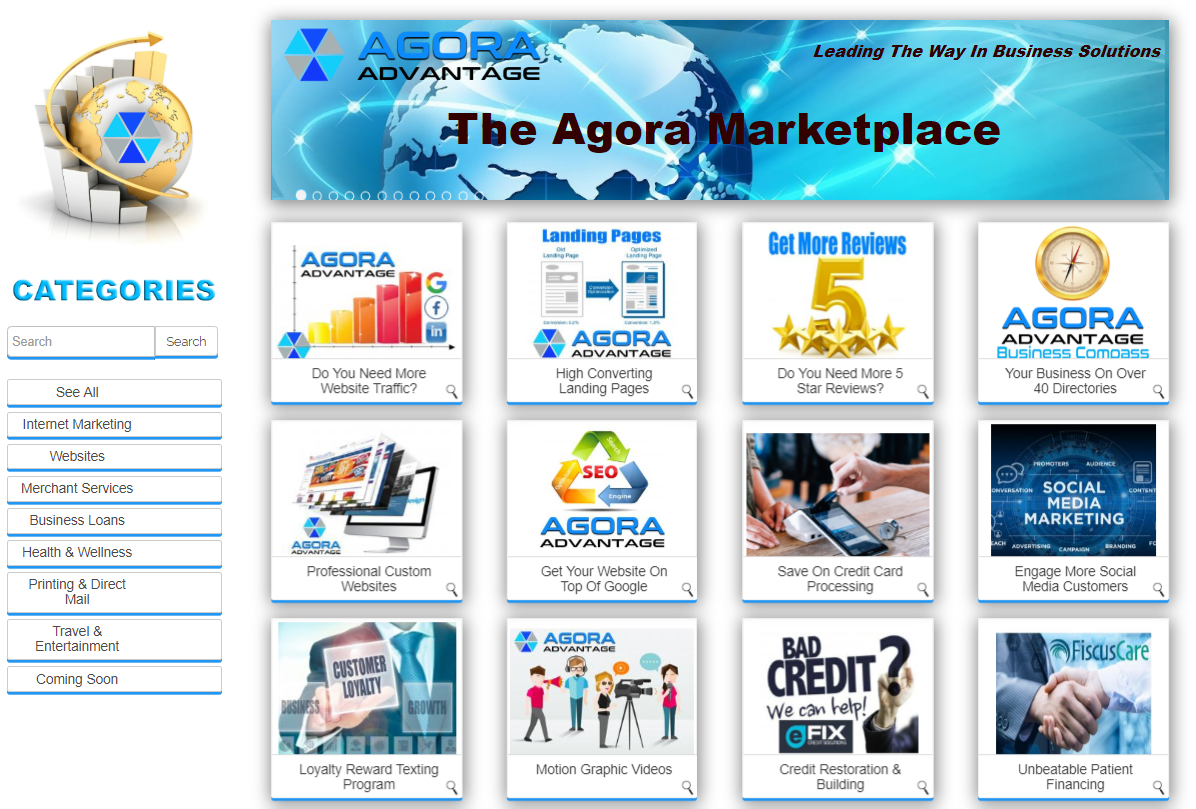This screenshot captures the homepage of a website named "Agora Advantage." At the top, there's a rectangular blue banner featuring a stylized blue and white planet. Superimposed on this image is the text, "The Agora Work Marketplace Leading the Way in Business Solutions."

On the left side, an illustration shows a planet ascending steps. The planet is depicted in yellow, white, varying shades of blue, and gray, functioning as a visual element for the "Categories" section. Below this, a search bar is present, followed by a list of categories: Internet Marketing, Websites, Merchant Services, Business Loans, Health and Wellness, Printing and Direct Mail, Travel and Entertainment, and a placeholder for "Coming Soon."

The main part of the page is divided into three rows, each containing four small boxes. These boxes showcase the various services offered by Agora Advantage, most of which incorporate the Agora branding. The services include:
1. "Need More Website Traffic?"
2. "High Converting Landing Pages"
3. "Get More Reviews"
4. "Agora Advantage Business Compass"
5. "Professional Custom Websites"
6. "Agora Advantage: Get Your Websites on Top of Google"
7. "Save on Credit Card Processing"
8. "Social Media Marketing"
9. "Loyalty Reward Texting Program"
10. "Motion Graphic Videos"
11. "Bad Credit Financing"

The boxes provide a comprehensive overview of the diverse business solutions Agora Advantage offers to its users.